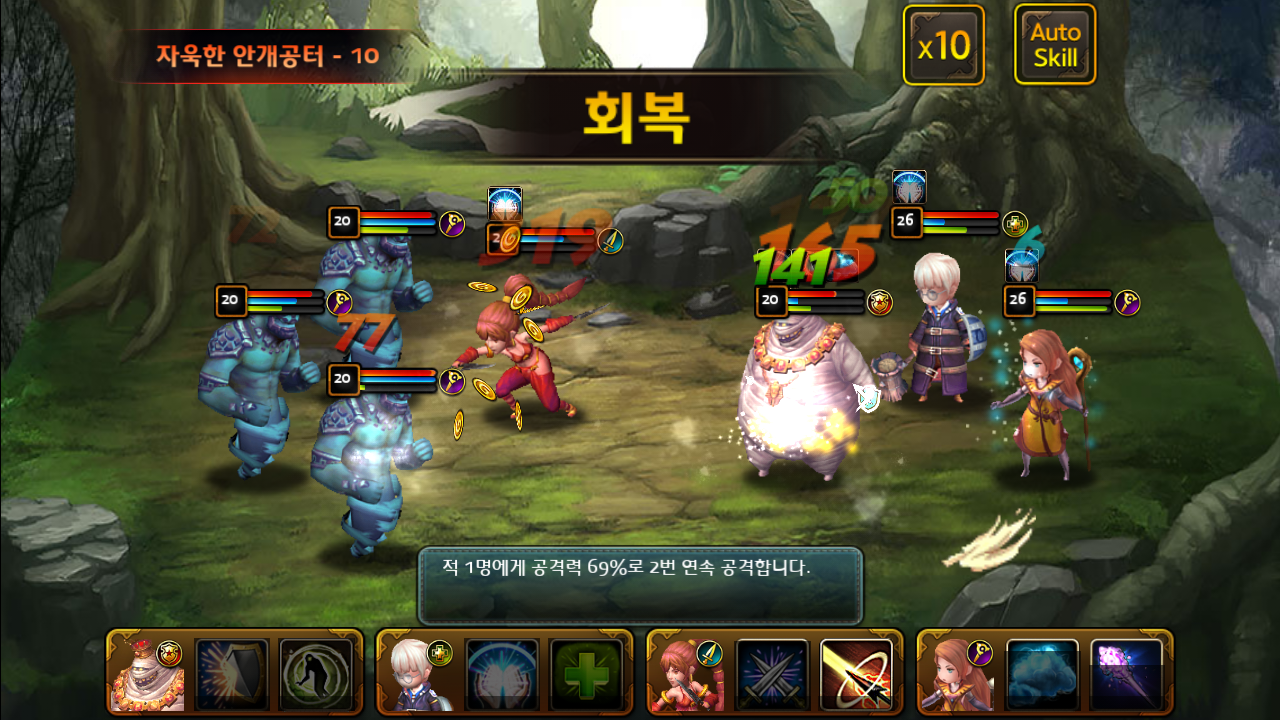This screenshot from a fighting video game showcases a dynamic battle scene set in a forest clearing, lit by incoming sunlight and framed by visible tree roots. Dominated by Japanese or Chinese characters, the image features two distinct teams. On the left, three blue ape-like ogres clad in shoulder armor, each marked with a score of 20, confront their opponents. One opponent, a red-haired girl with pigtails wearing red pants and wristbands, is hurling what appear to be gold coins at the blue ogres, with a score of 2 above her head. On the right, a diverse trio stands ready: a large smiling ogre adorned with a glowing gold necklace, a young blonde boy in a blue buckled outfit, and a brunette girl surrounded by blue sparkles, suggesting magical abilities. The scene blends anime and computer game art styles, creating a vibrant and engaging visual narrative.